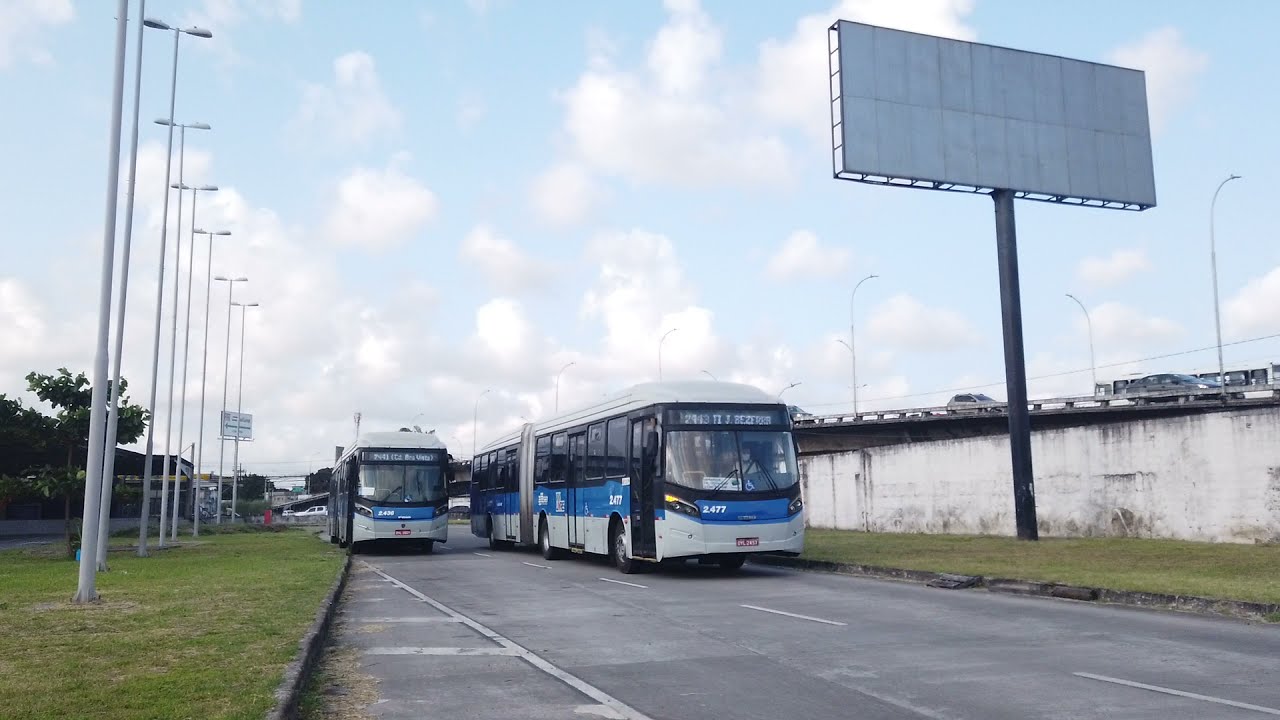The image is a detailed color photograph taken on a partly cloudy day, depicting a scene with two public transport buses traveling on a paved road towards the bottom right. Both buses are white with a distinctive blue banner running along the sides and front. The bus on the right is slightly closer to the viewer, marked as bus number 2477, while the one on the left is positioned a bit farther back, making its number illegible. The buses feature overhead message boards with unreadable text above the driver's windows.

The road is flanked by grassy areas. On the left side, there is a row of tall white streetlights, currently turned off, extending into the distance. On the right side of the roadway, elevated slightly, a secondary road can be seen with cars driving along it. A billboard with a blank face, mounted on a long steel pole, stands near a white parking structure with a guardrail atop it behind the buses. The sky occupies the upper two-thirds of the image, showcasing a large expanse of blue interspersed with white, fluffy clouds. The overall visual style of the photograph is realistic, typical of representational realism.